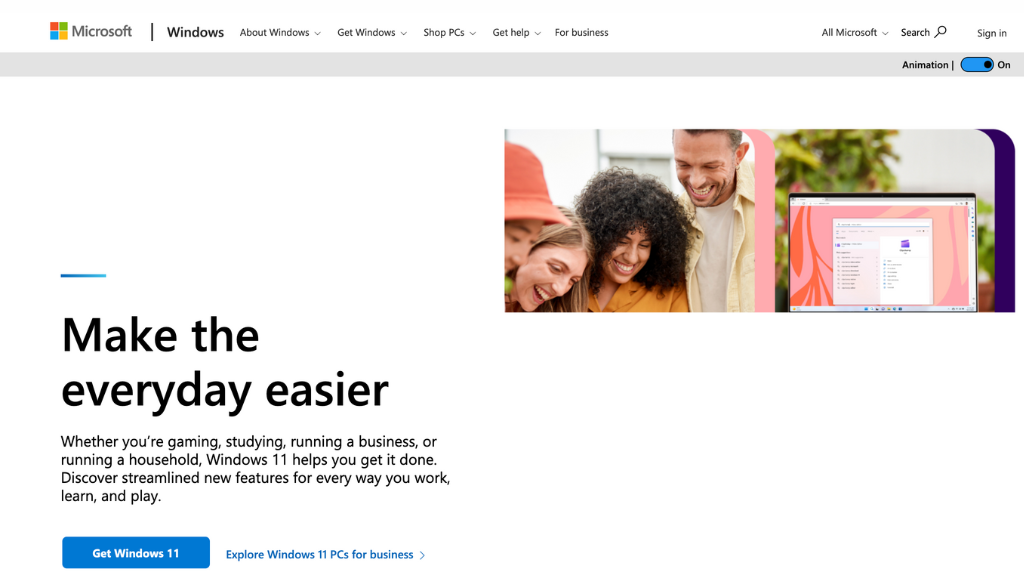This is a detailed screenshot of a website primarily showcasing Microsoft's Windows. The header is white and features the Microsoft logo on the left, composed of four multicolored squares: blue at the bottom left, red at the top left, green at the top right, and yellow at the bottom right. To the right of the logo, "Microsoft" is written in gray sans-serif text, followed by a vertical black separator line, and then "Windows" in black text. To the right of this, there are several menus in gray text labeled "About Windows," "Get Windows," "Shop PCs," "Get Help," and "For Business," each with a downward-pointing arrow.

On the far right of the header, there is an "All Microsoft" menu with a downward-pointing arrow. Next to it is a black search label with a black magnifying glass icon, followed by a small area of negative space and gray text that reads "Sign in."

Beneath this header, there is a light gray sub-header that is largely empty, except for a couple of items on the right side: bold black text that reads "Animation," a vertical black separator line, and a blue selection button with a black outline and black text that reads "On."

The body of the web page has a white background. In the top right, there are two photographs: one on the left shows four people leaning together and smiling, and the one on the right displays a blurred plant with a screen superimposed over it featuring a pink and red background with a black header. Colorful stripes appear to the right of each image, with pink on the left photo and purple on the right photo, both curving upward to the left.

Beneath the images and on the white background, large black text reads "Make the everyday easier."